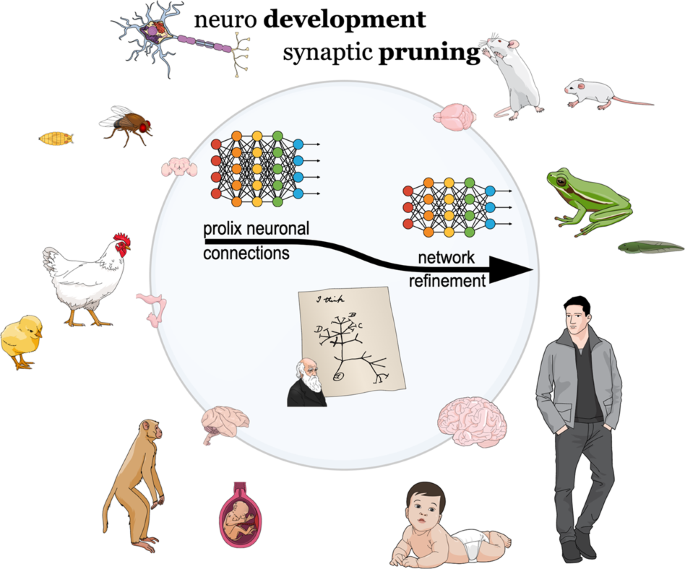The image is a detailed, digitally-created diagram illustrating neurodevelopment and synaptic pruning, with the text "Neurodevelopment, Synaptic Pruning" prominently displayed in black at the top against a white background. The central circle features interconnected black lines denoting Proleg's neuronal connections and network refinement. Surrounding this central concept are various organisms and developmental stages, presented in a circular arrangement. From a small insect and a cockroach to a hen and chick, two white mice, a green frog, an embryo or monkey, and culminating in a baby and an adult man dressed in a grey outfit with an increasingly larger brain, the diagram visually represents the evolutionary stages and complexity of brain development. Additionally, there is an image of Charles Darwin with a related diagram or equation at the bottom, reinforcing the evolutionary theme. The overall color palette includes black, grey, green, red, yellow, blue, off-white, and pink, and the layout and design convey a scientific, educational focus on neurodevelopment.